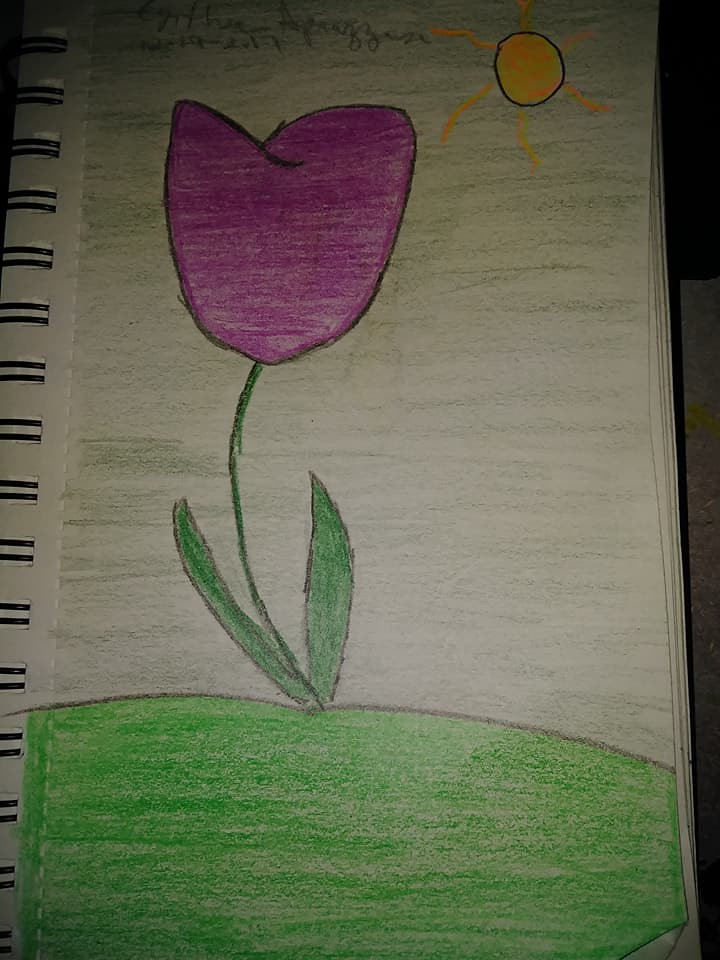This is a color photograph depicting a child's simple line drawing created on a piece of white notebook paper. The photograph appears to have been taken indoors under poor lighting conditions, making it difficult to discern fine details. The notebook paper features a dark binding on the left edge of the right-hand page visible in the image. To the right edge of the paper, a darker, possibly wooden surface can be seen beneath the notebook, along with the edges of numerous other pages.

At the top of the drawing, there is some pencil writing that is unreadable—potentially a signature or a brief explanation of the artwork. Evidently, the drawing was initially sketched in pencil and later colored with dark pencil shades.

Prominently featured in the center of the page is a tulip, characterized by an oval-shaped flower head filled in with a deep pink hue. The tulip's stem is thin, accompanied by pointed leaves, both of which are shaded in green. Underneath the tulip, green grass is sketched with dark pencil outlines and subsequently filled in with green color.

The background exhibits pencil strokes in a greyish-green tone, adding depth to the scene. In the upper right-hand corner of the page, a sun is illustrated. It is outlined by a dark pencil circle and filled with yellow, accented with orange-yellow sections. Radiating from the sun are spiraling lines in varying shades of orange and yellow, symbolizing sun rays.

Overall, the image captures the whimsical and creative essence of a child's drawing, with vibrant colors and thoughtful details that bring a simple tulip and sunny day to life.